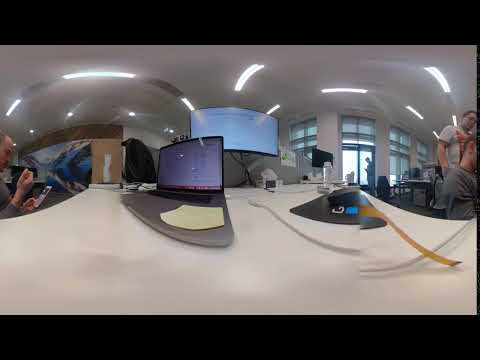The image portrays an office-like environment with various objects and people arranged meticulously. Central to the scene is a white table occupying the bottom half of the image, on which sits a gray laptop with a black keyboard located towards the left. To the right of the laptop, a piece of paper is visible. Seated at the table on the left side, a balding man in a gray long-sleeve shirt is focused on something in his hands. Adjacent to him are two other individuals; one in a light gray t-shirt is seated, and another in a white t-shirt stands looking over his shoulder. Above the table, a TV with a blue screen is mounted on a light brown wall. In the background to the right, another TV with a black screen is seen along with windows letting in natural light. The ceiling, at the top of the image, features distinctive fluorescent lighting casting a whitish-yellow glow. The image also includes details such as the white borders around the TVs, creating a contrast with their dark screens. The setting suggests a work-related or administrative space, enhanced by elements like a yellow notepad and the overall structured arrangement of objects and people.